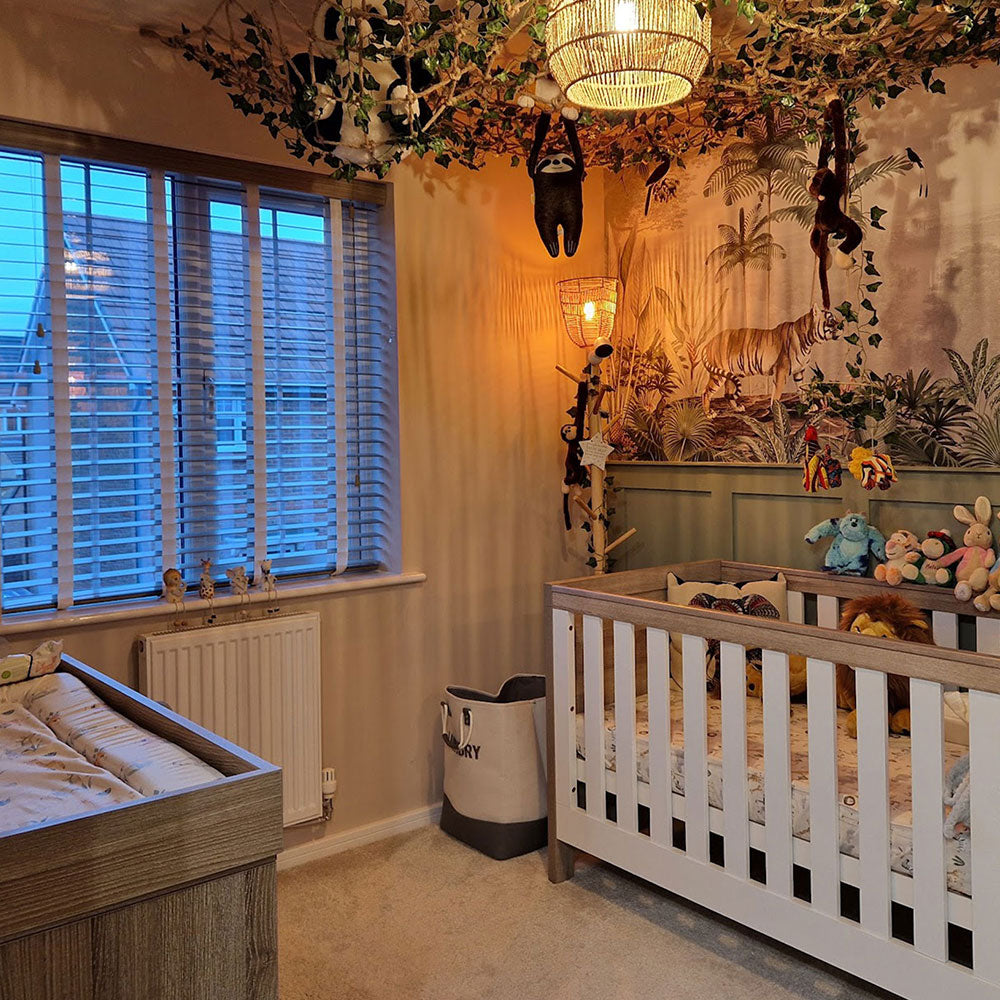The image captures a vibrantly decorated nursery with a distinct jungle theme. Dominating the right side of the room is a white crib accentuated with wooden brown trims, featuring a patterned mattress. The crib is adorned with an assortment of stuffed animals, including bunnies, characters from Monsters Inc., Tigger, and various dinosaurs. Surrounding the crib are more stuffed animals like a lion, a tiger, and a bunny rabbit. 

The nursery walls are painted with jungle scenes, displaying a variety of animals and plants such as tigers, cats, ferns, and tall grasses. Above the crib, a sophisticated light fixture resembling tree branches hangs from the ceiling, adorned with sloths, pandas, and monkeys. Adjacent to the crib on the left is a changing table, and a window with wooden blinds adds natural light. The window is complemented by netting and fake plants to enhance the jungle atmosphere, along with a whimsical monkey and a panda hanging from the net.

Additional details include a white heater beneath the window and a bag placed next to the crib. The color scheme predominantly features tans and browns, contributing to the warm, jungle-like ambiance of the nursery.